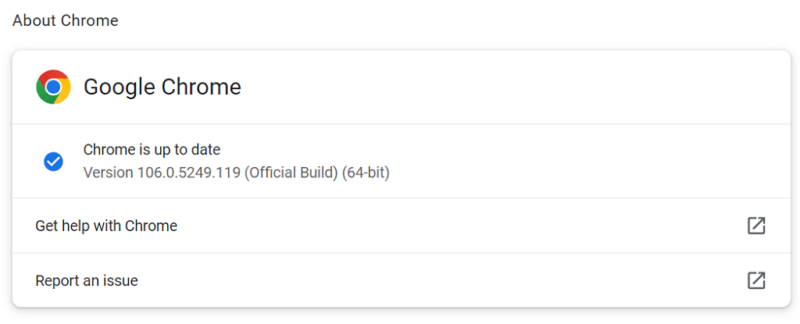This image depicts a webpage about Google Chrome with a clean, white background. The main content of the page is centered inside a bordered section, while an introductory text titled "About Chrome" is positioned outside of this bordered section, in the top-left corner.

In the main section, the information is presented in four distinct rows. At the top, the text "Google Chrome" is prominently displayed next to the Google Chrome icon, which is a circular symbol featuring the colors green, red, yellow, and a blue inner circle outlined in white.

Below this header, a message indicates: "Chrome is up to date," followed by specific version details: "Version 106.0.5249.119 (Official Build) (64-bit)." To the left of this message, there is a blue-filled circle icon with a white checkmark inside it, signifying that the application is current.

Further down, a section titled "Get Help with Chrome" appears, accompanied by a gray square icon with an arrow pointing to the top right on its right side, suggesting a link to additional resources or support.

At the bottom, the page also includes an option to "Report an Issue," which is similarly accompanied by a gray square icon with an arrow pointing to the top right, indicating this is also a clickable link.

The overall theme is minimalist, with a focus on providing essential information about the browser's status and functional support options against a clear, white backdrop.